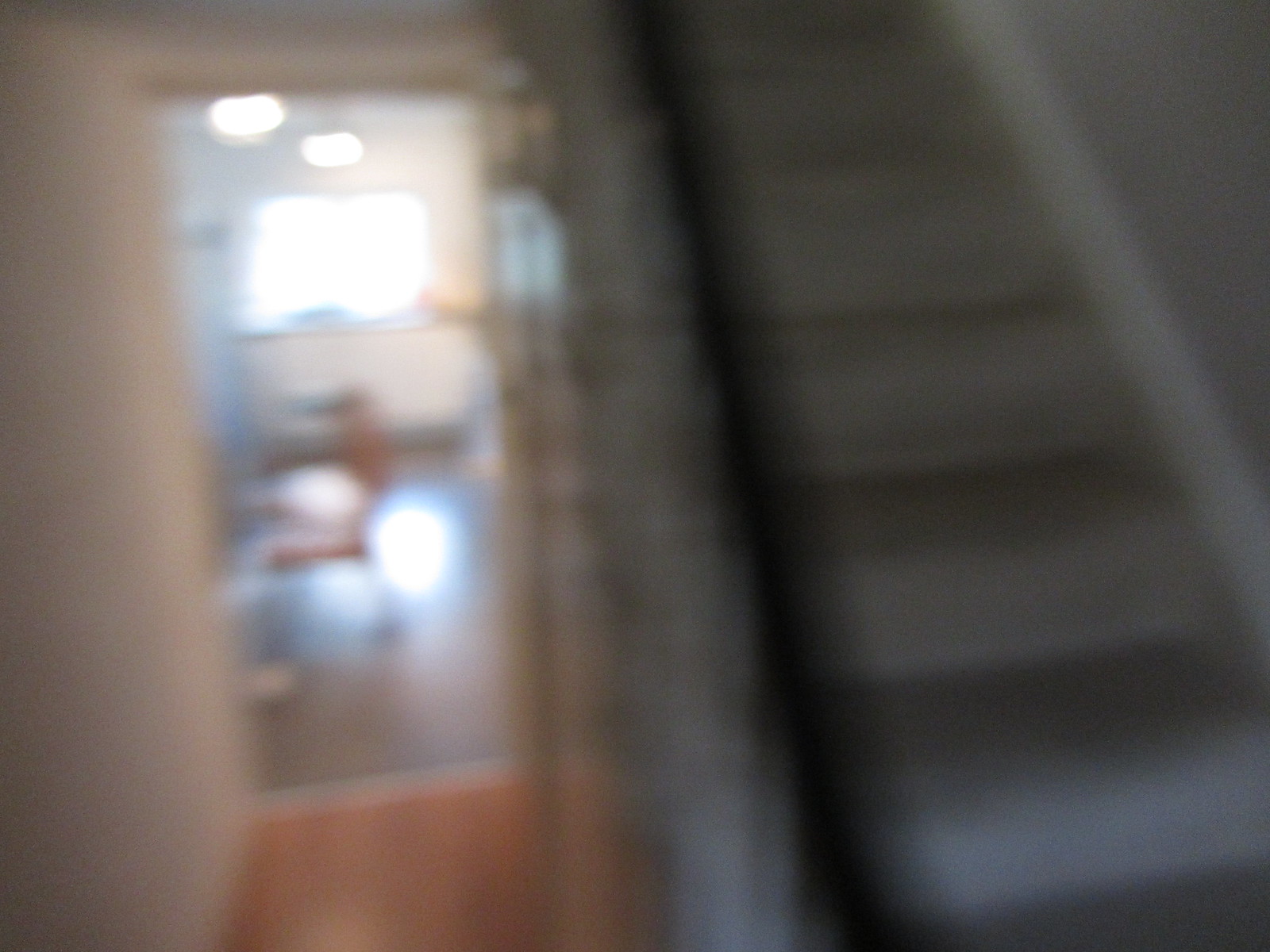The image is a blurry digital photo capturing the interior of a house, possibly taken from a foyer or hallway that leads into a kitchen. On the left side of the photo, a white wall is visible, while the right-hand side is dominated by a staircase ascending vertically. The staircase features a darker handrail, likely black, and white banisters, with a white skirting board running alongside and a grey wall in the background. The stairs are carpeted in a creamish tan color. The floor of the hallway appears to be a lighter brown laminate or wood, transitioning to a darker brown or greyish flooring in what is assumed to be the kitchen area. This transition is marked by a doorway with a white frame. In the kitchen, there's a yellowish chair visible, pushed in with its back facing the viewer. A square window on the back wall lets in substantial natural light, and two white ceiling lights are also on. The image, though extremely blurred, also shows some glare on the floor, indicating a shiny, perhaps laminate surface. Overall, while the photo is fuzzy, the basic layout and key elements like the staircase, doorway, and kitchen can be discerned.